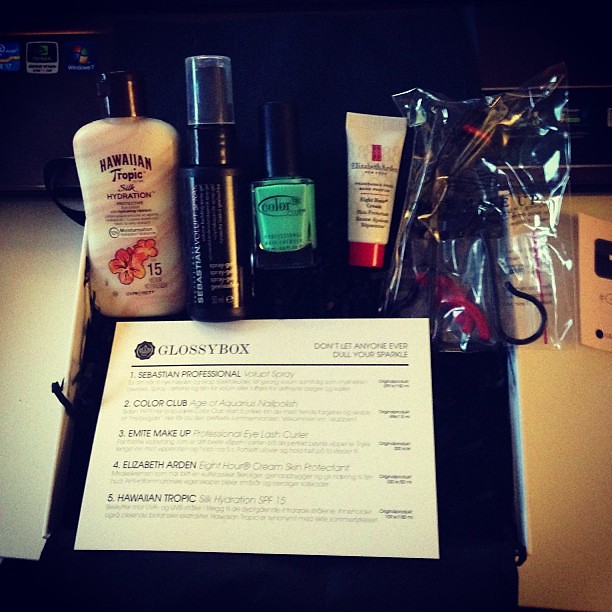In this detailed image, a variety of cosmetic products are neatly arranged on a white desk with a black background. At the bottom of the image, a white card labeled "Glossy Box" describes the items. The first item on the left is a tan plastic bottle of Hawaiian Tropic Silk Hydration sunscreen with SPF 15, featuring an image of hibiscus flowers and a dark brown cap. Next to it is a black spray bottle of Sebastian Professional Volupte hairspray with a translucent cap. Following that is a bottle of sea green nail polish by Color Club, with a square shape and a black cap. Beside it is a small white tube of Elizabeth Arden skincare cream with a red cap. Finally, a pair of eyelash curlers can be seen in a reflective cellophane bag.